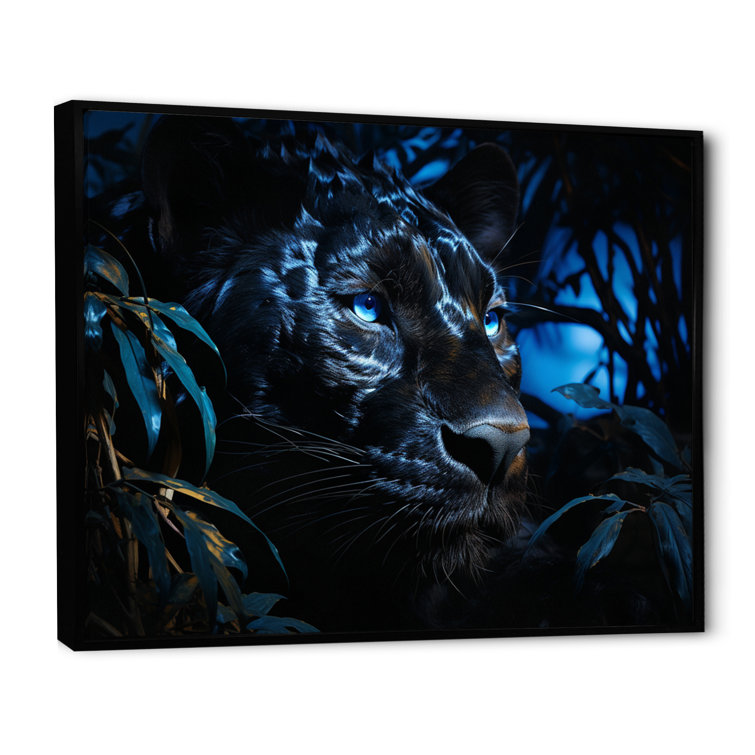The image is a canvas painting featuring an exquisitely detailed, dark-colored tiger amidst a shadowy jungle setting. The composition is notably somber, dominated by hues of black and midnight blue, with streaks of dark brown and light blue intricately woven throughout the tiger's face. The focal point is undoubtedly the tiger's head, which appears illuminated by a subtle blue moonlight, lending a glossy sheen to certain areas of its dark fur. The tiger's piercing light blue eyes, with black pupils, draw immediate attention, offering a stark contrast to the surrounding darkness.

Around the tiger's face, tropical foliage adds to the jungle ambiance. On the left-hand side, dark green leaves create a silhouette against the black background. The right-hand side features plants with a lighter bluish-green tint, accented with subtle yellow hints at the base, all illuminated by the mystical blue light. The presence of the blue moon distantly adds a surreal and otherworldly atmosphere to the scene. The tiger's black nose and discernible whiskers further enhance the realism and depth of the painting, making it a captivating focal point of any space.